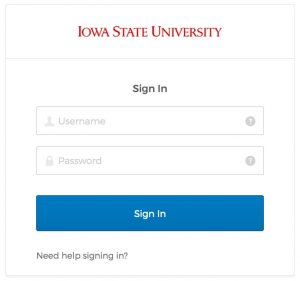This image captures the sign-in screen for Iowa State University. At the top, within a white box outlined in a thin gray line, the university's name, "Iowa State University," is prominently displayed in red. Below this header, the screen presents the login interface, starting with a user name input field followed by a password field. Beneath these input fields, a blue "Sign In" button invites users to access their accounts. For those experiencing difficulties with the login process, a gray text link positioned at the bottom offers assistance, stating, "If you need help signing in, click here."